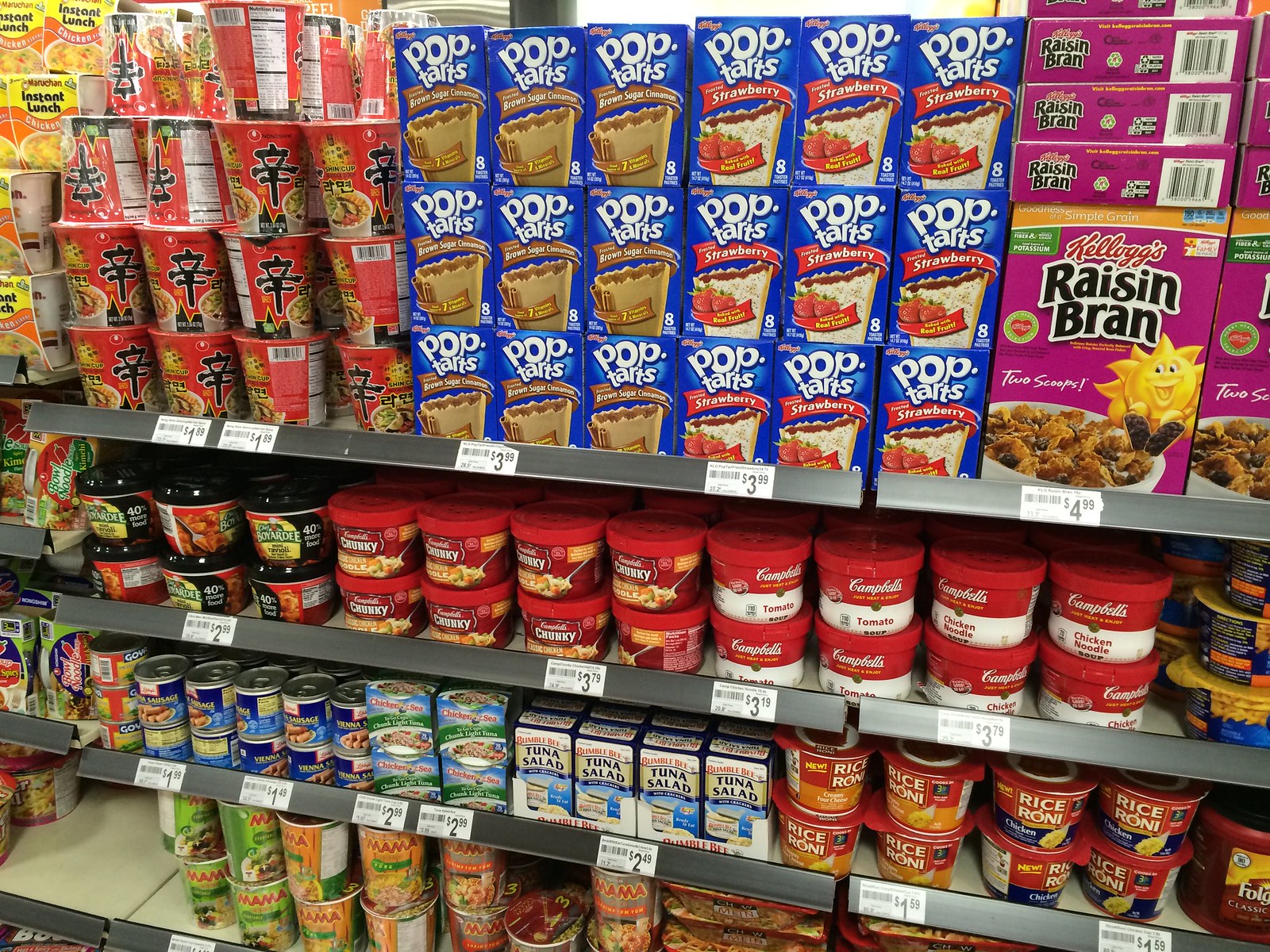This image depicts the interior of a well-stocked supermarket aisle, viewed from the perspective of a shopper browsing a line of shelves. 

Starting from the top shelf, there are rows of Pop-Tarts in two flavors: strawberry and brown sugar. To the upper right of the Pop-Tarts, a neat arrangement of Raisin Bran cereal boxes is clearly visible. On the left of the Pop-Tarts, a variety of Asian brand noodle cups are prominently displayed, ready for quick and convenient meals.

The second shelf down features an assortment of microwavable containers of popular Campbell's soups, including both the classic and Chunky varieties, along with Chef Boyardee products.

The third shelf below showcases a selection of ready-to-eat Tuna Salad from Bumble Bee, various flavors of Rice-A-Roni, and cans of Vienna Sausages by Libby’s, catering to a variety of taste preferences and meal options.

The bottom shelf is dedicated to a brand called Mama, with all items neatly organized in cans, completing the diverse array of food products available in this supermarket aisle.